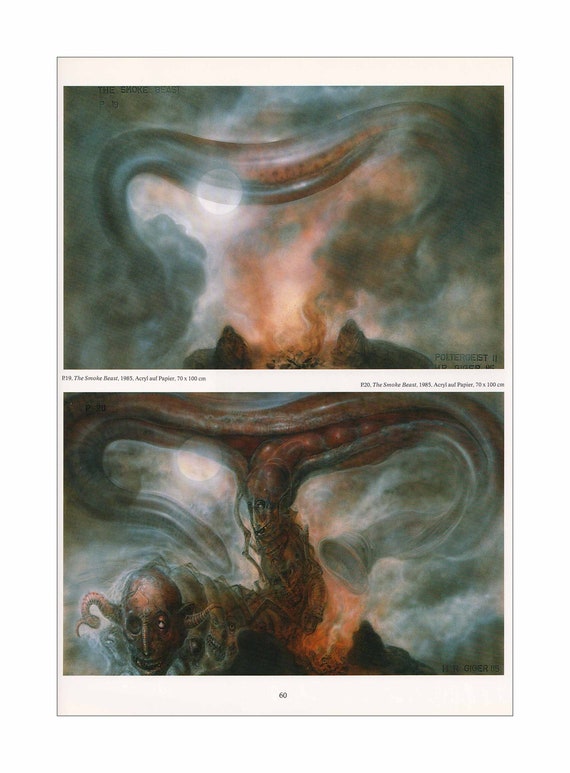The image consists of two paintings presented vertically, each portraying different but related eerie scenes linked by the theme of a "Smoke Beast." The top painting, labeled "R-19, the snake beast, the smoke beast, 1965, acrylic and paper, 70 by 100 centimeters," features a smoky, serpent-like figure rising from the center of a campfire where two blurred individuals sit. The serpent’s body is composed of dark gray and brown hues, merging naturally with the swirling smoke. Its form is indistinct, lacking a defined head or tail, which enhances its ghostly presence. There is also a subtle depiction of a moon adding to the mystical atmosphere.

The bottom painting, marked as "P-20, the smoke beast, 1985, acrylic and paper, 70 by 100 centimeters," maintains the same medium and dimensions. This painting showcases a central campfire from which smoke forms a demonic figure. The figure’s face is zombie-like, with one missing eye, pronounced pointy ears, and horns. Additional smaller demonic heads cascade inward toward the fire and spread outward, intertwining into elaborate horn and smoke formations. The color scheme remains consistently dark with predominant brown and gray tones, conveying a foreboding and supernatural ambiance. Both pieces of art evoke a sense of connection to the ethereal 'Smoke Beast,' blurring the boundaries between reality and the paranormal, much like a scene from a vintage horror story.